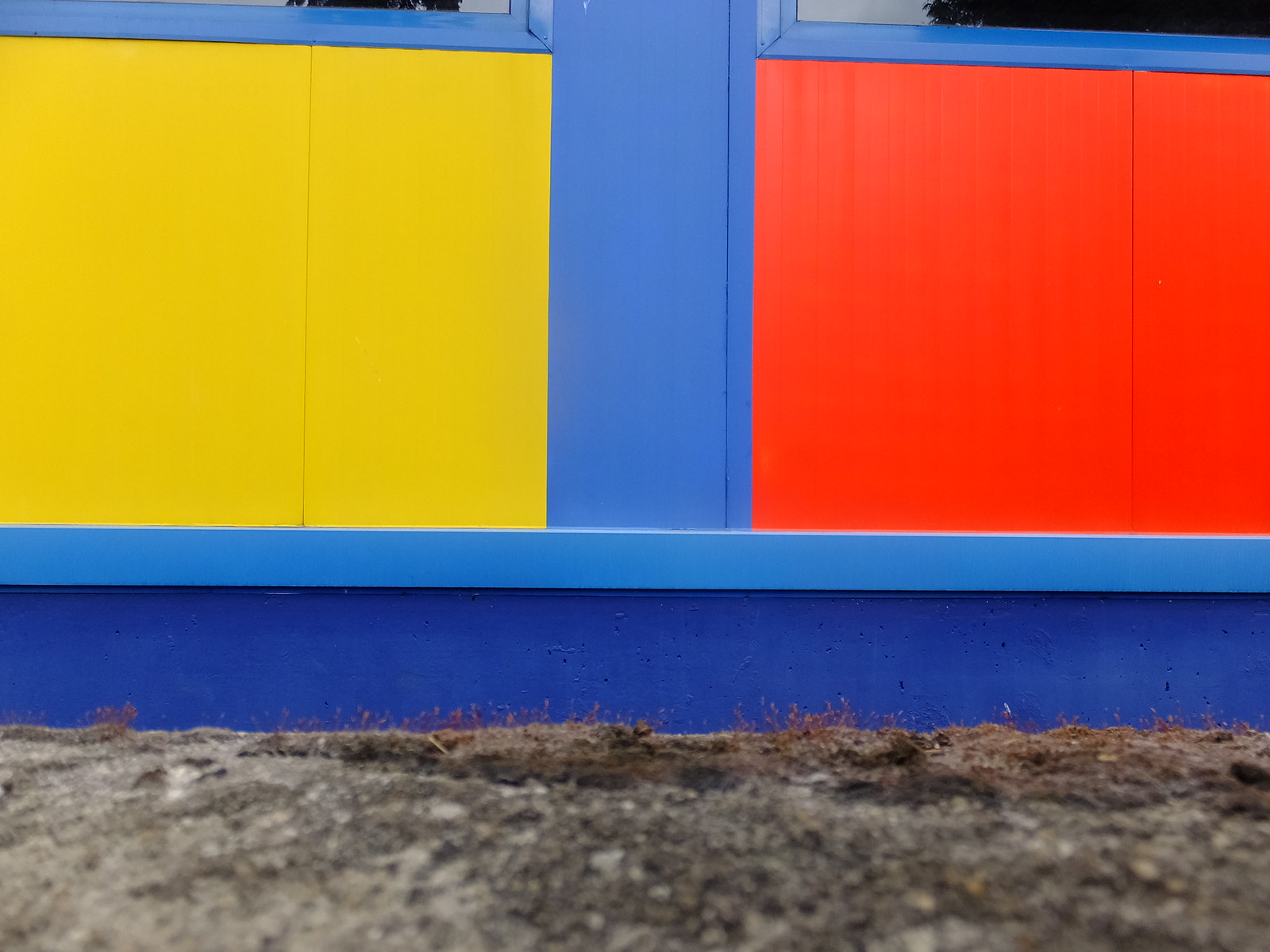In this daytime photograph, we see the side of a building featuring a striking painted wall. The left portion of the wall is bright yellow, while the right side exhibits a vivid red. These colorful sections are bordered by a deep blue area, creating a visually engaging contrast. Situated above these painted sections are windows, visible only at their bases. The bluish reflections in the windows hint at a grayish sky and some background trees. Below the wall, the ground consists of sandy, grayish dirt interspersed with brown patches and sparse, dried weeds, indicating a neglected or perhaps wild state. The dark blue baseboard of the wall, slightly recessed, adds another layer of depth and detail to this visually arresting composition.